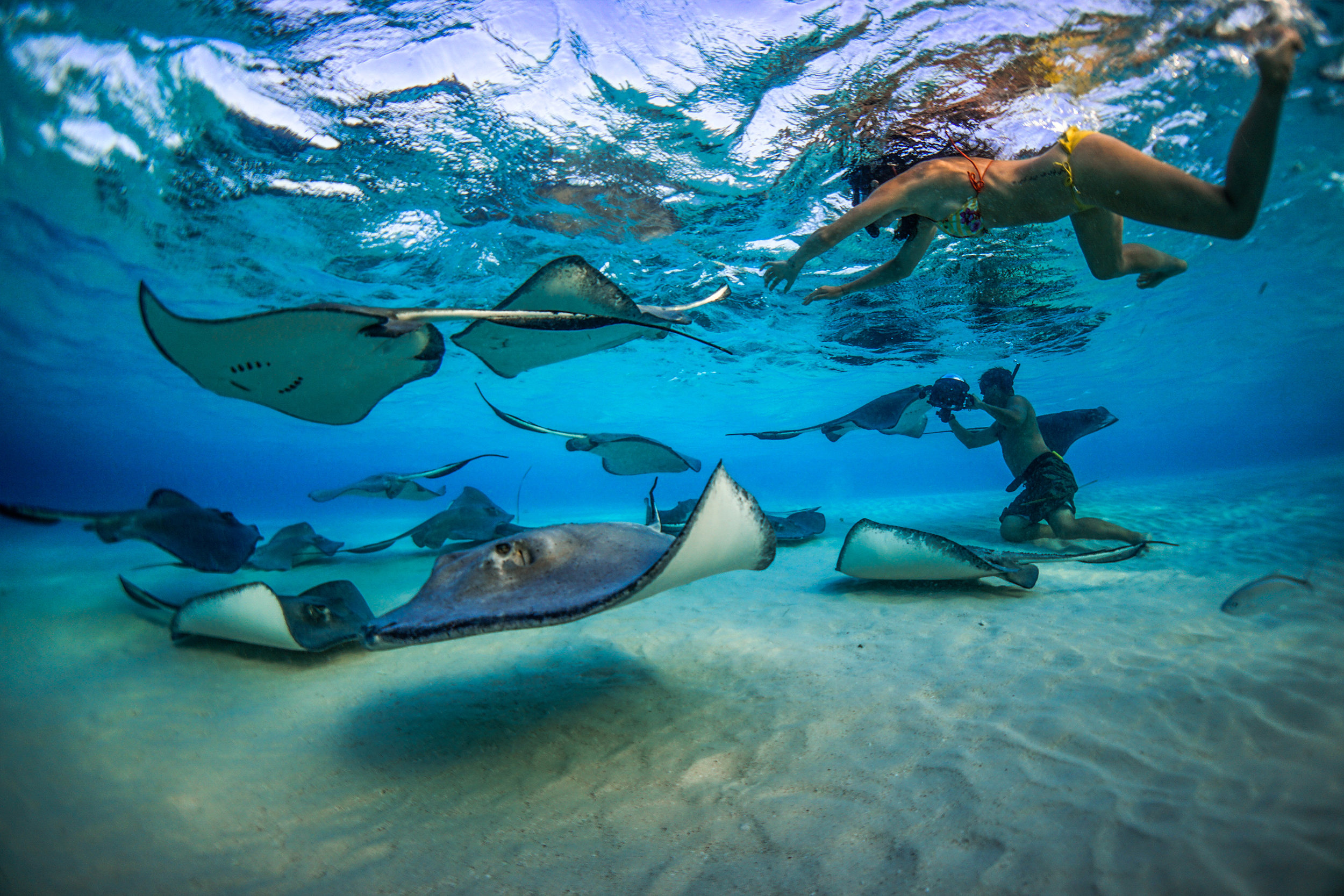In this underwater photo, we're immersed in a world of beautiful, crystal-clear turquoise water. The bottom of the scene is covered with white, powdery sand, and the sunlight dances through the water, creating ripples and shadows on the sand below. Numerous stingrays of varying sizes and shades of gray are gracefully gliding through the water, some close to the surface and others near the sandy bottom.

Two people are interacting with the stingrays. A woman in a bikini, with a red top and yellow bottoms, is just below the surface, reaching out towards one of the stingrays. She appears to be floating effortlessly in the clear water. Meanwhile, a man, who is wearing just shorts, is closer to the sandy seabed. He seems to have a camera or video camera in hand, possibly capturing the enchanting scene, with his knees touching the sand. Both individuals are equipped with scuba or snorkeling gear, fully immersed in this serene underwater landscape.